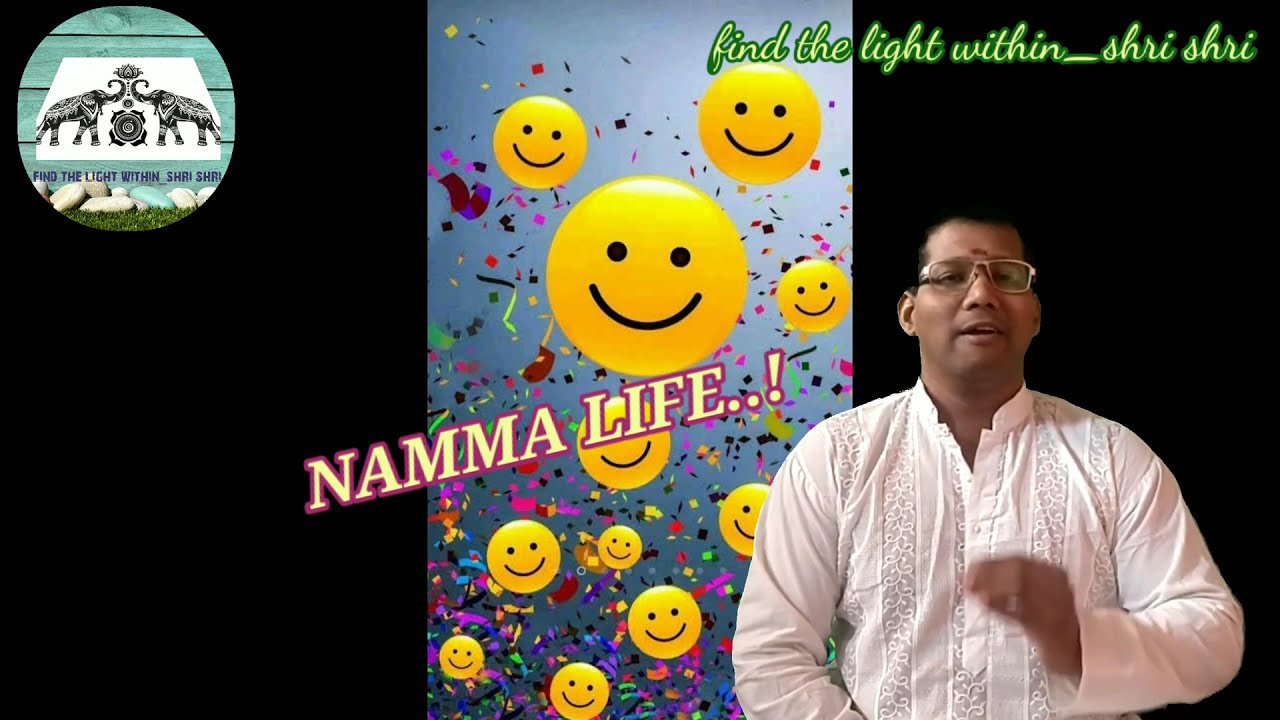The image is a rectangular, three-part composition comprising various elements and rich in detail. In the upper left section, set against a turquoise background with horizontal wood planks, a round emblem features two elephants facing each other under a lotus flower, with a circular symbol beneath them. Below the emblem, white text reads, "Find the light within Sri Sri." A mixture of white and turquoise stones, along with green grass, complements this area. Moving to the center, a vertical blue background is adorned with colorful confetti and numerous smiley face emojis. Overlaid in the middle, the text "Namma Life.." in white with a pink outline adds a vibrant touch. The right section captures a South Asian man with short black hair and light brown skin, wearing a traditional white shirt with embroidered panels and white-framed glasses. The man, appearing in mid-speech with one hand raised, is framed by a black background. The cursive green text, "Find the light within Sri Sri," is prominently displayed above him. The image combines cultural motifs, celebratory elements, and an animated human subject for a visually engaging and narrative-rich composition.